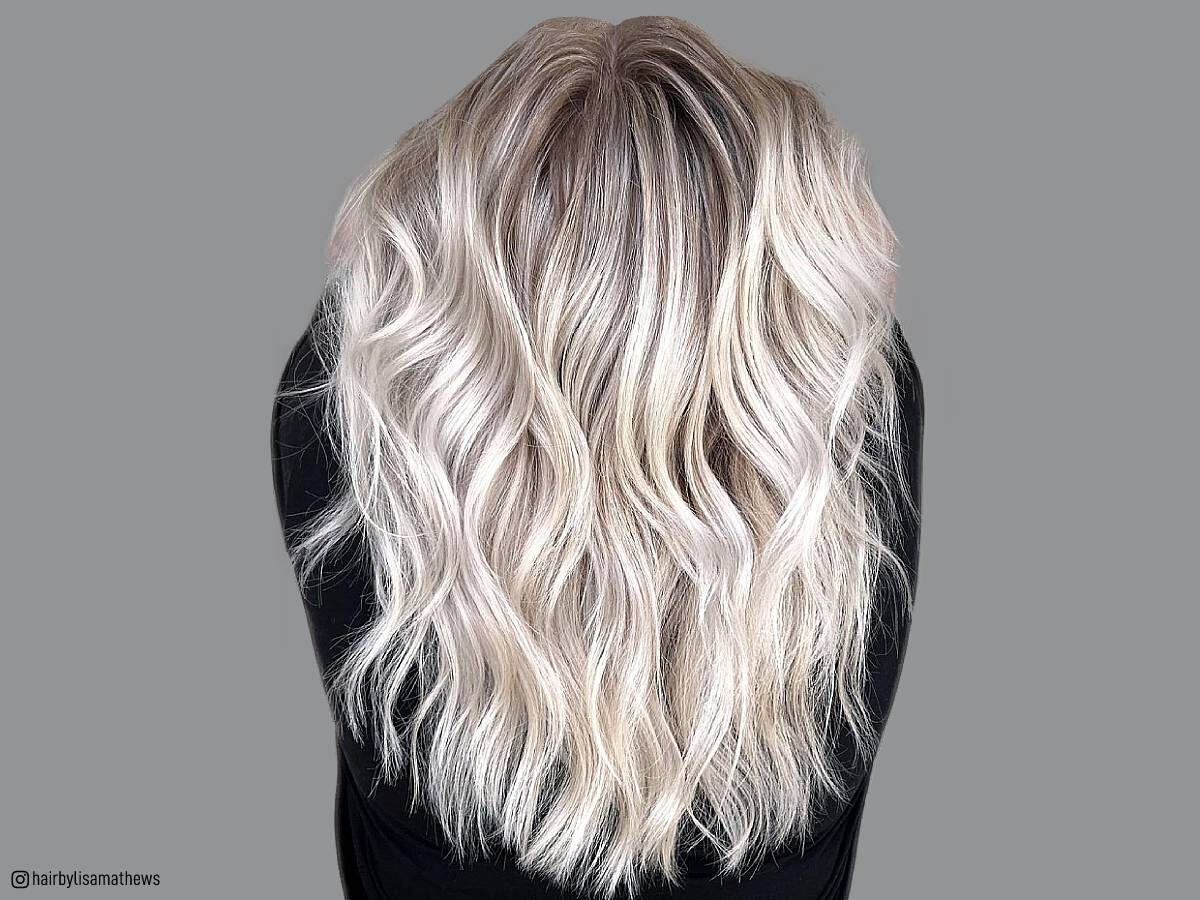The image showcases the back view of a woman's newly styled hair, presumably taken as an advertisement to highlight the expertise of a professional hairstylist. Set against a flat gray background, the woman's shoulder-length hair features a striking blonde balayage that transitions seamlessly from darker roots at the top to increasingly lighter, silvery blonde strands toward the bottom. Her wavy and slightly curled hair appears remarkably shiny and voluminous. She is dressed in a long-sleeved black top. Notably, the bottom left-hand corner of the image features the black text "hair by Lisa Matthews," emphasizing the work of the hairstylist.